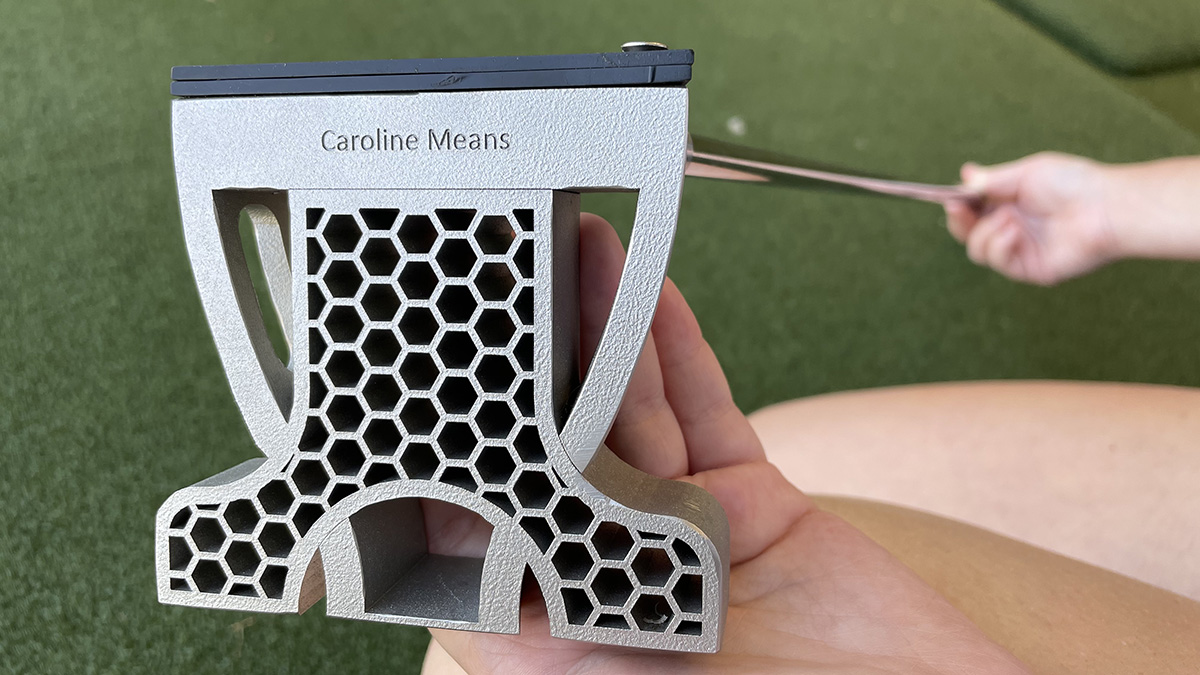This highly detailed image captures a unique metallic object, resembling an award or an unusually designed golf putter, held by two hands against a green background, possibly artificial grass. The main structure is visually intriguing, composed of a dual form: an outer V-shaped frame that somewhat mimics the shape of a cup, and an inner segment forming a Y-like assembly with several large, hexagonal honeycomb cutouts. The object's metallic surface is predominantly silver, but it features a contrasting blue strip towards the top. The item bears the inscription "Caroline Means" on its upper side. One can see a nail protruding from the top-right corner and the person displaying the object appears to have a white complexion. The photo's angle is from above, focusing closely on the object, causing the shaft or handle part to blur into the distance towards the right. The well-lit scene enhances the object's intricate metal construction and the background provides a natural, yet clearly staged context for the image.